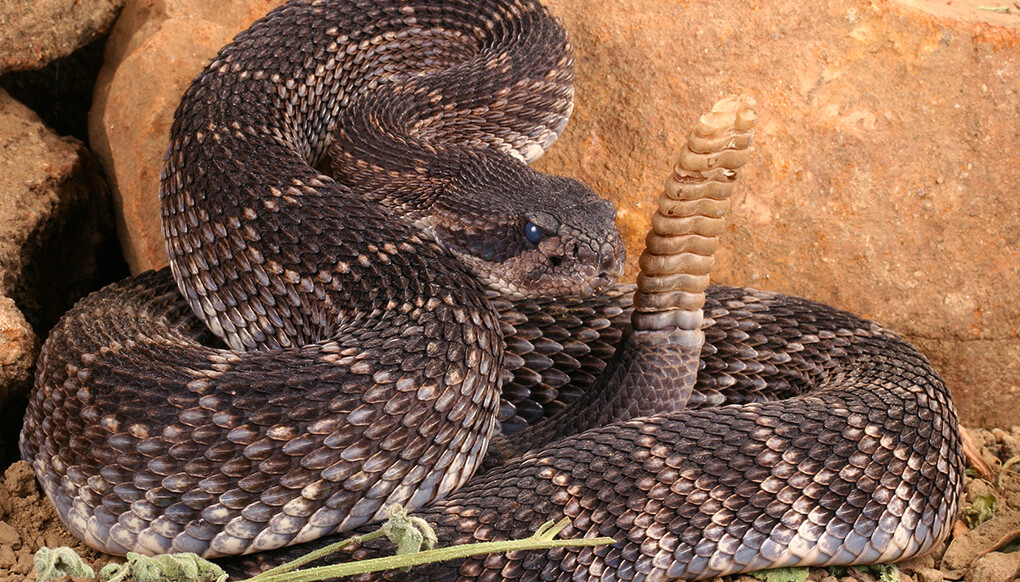This close-up image captures a fierce-looking rattlesnake coiled up against a background of reddish-brown rocks. The snake, occupying nearly the entire frame, has its tail—with a distinctive rattle—sticking up prominently in front of its face, almost as if it is staring at its own rattle. The rattlesnake's scales are dark brown to black with interspersed lighter patterns of whites, creams, and grays, and a prominent black stripe runs from its head to its tail. The lighting and setting suggest that the photo might have been taken in a controlled environment like a zoo exhibit rather than out in the wild. The rocks and a small green plant at the bottom left corner enhance the naturalistic appearance. The snake's blueish eye is fixed intently, giving it an alert and aggressive demeanor, ready to strike.